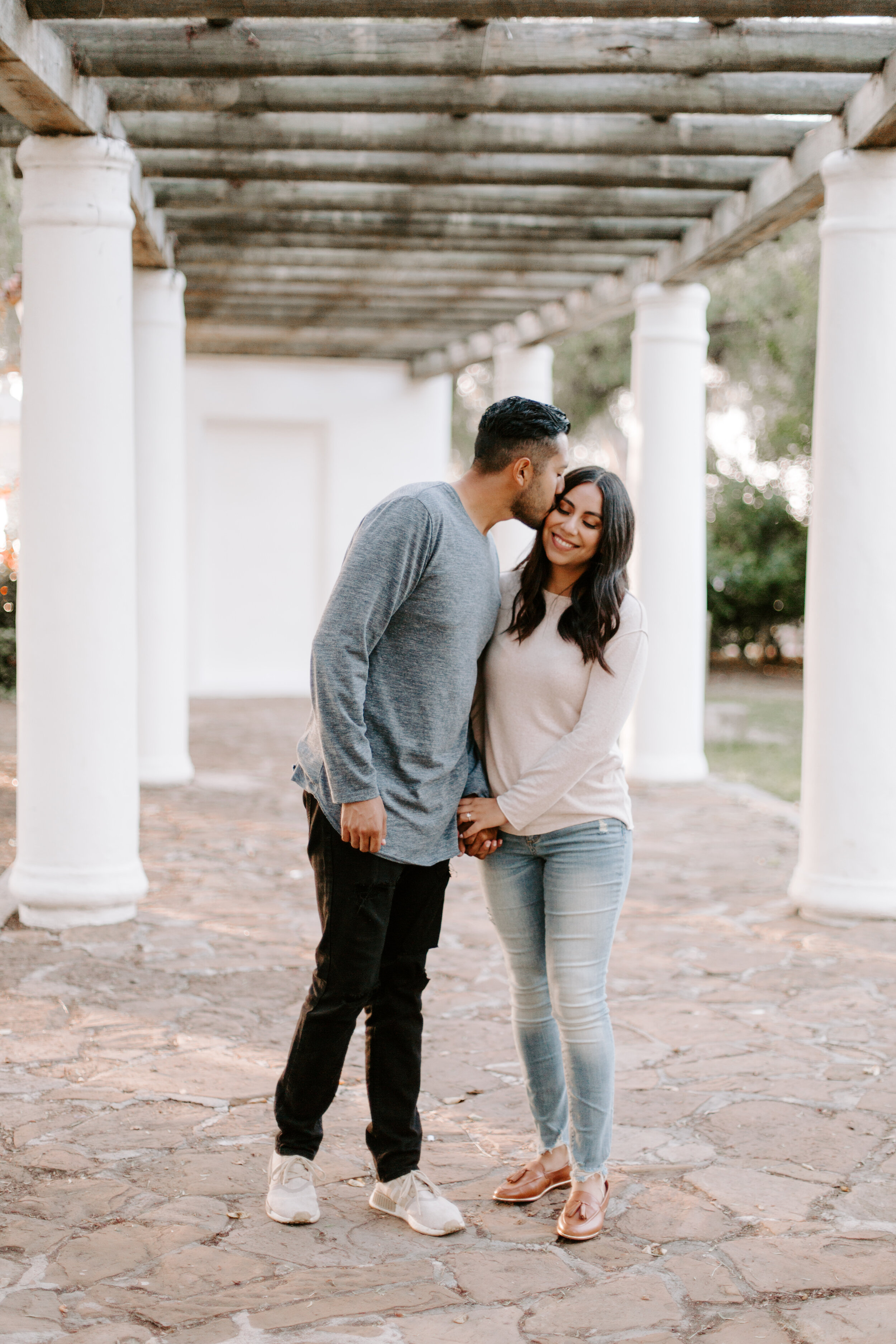In this photograph, a young couple, possibly in their late 20s or early 30s, stands at the center of an outdoor setting that appears to be under a veranda. The area features a cobblestone pathway in tan and white hues. They are surrounded by four large white pillars supporting a distressed wooden ceiling with industrial-style beams. In the background, there is also a white wall with visible branches and leaves, giving a partial view of trees and creating a serene natural ambiance.

The man, who seems to have a faded haircut and possibly of Indian or Spanish descent, is dressed in a long-sleeve gray shirt, black fitted pants, and white sneakers. He has short black hair and some facial hair, and he is leaning down to kiss the side of the woman's head. The woman, with long wavy black hair, is smiling with her eyes closed, embracing the moment. She wears a cream-colored long-sleeved top, light-washed jeans, and tan loafers with tassels. She holds the man's left arm with both of her hands, adding a tender touch to the romantic scene, which could easily be part of an engagement shoot.